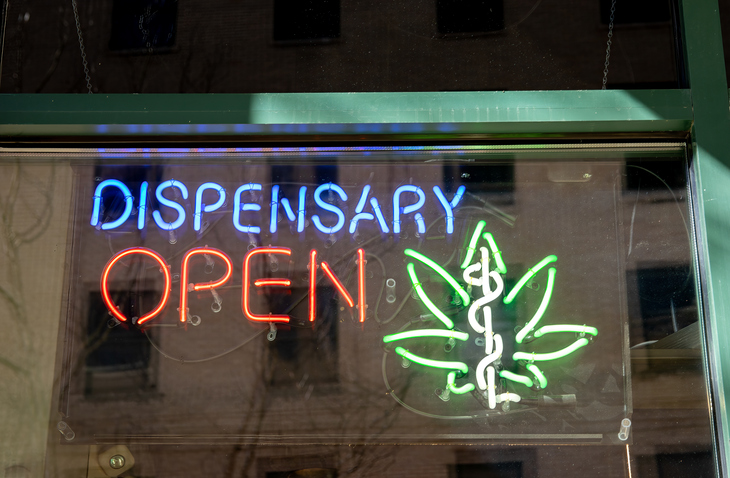This photograph captures a marijuana dispensary store window featuring a neon sign that prominently announces "dispensary" in blue text and "open" in red text. To the bottom right of the sign, a green marijuana leaf with a white medical caduceus symbol through its center stands out, forming the logo. The neon sign, which is suspended by chains, is set against a clear glass window, bordered by a green-painted frame. Reflected in the glass is a large, multi-story brick building with several dark windows, adding depth to the scene. Additionally, faint reflections of wires or vines seem to hang down along the left side of the window, further contributing to the urban setting.